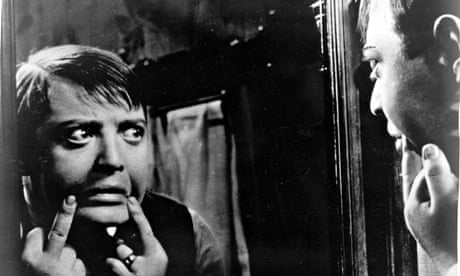This black-and-white photographic still shot from a movie features the renowned actor Peter Lorre in an intense, macabre scene. The setting appears to be indoors, with a meticulously framed composition that underscores the dramatic tension. In the top right corner, a partial image of Lorre's face can be seen, echoing the expression of the larger, more dominant figure in the bottom left corner. 

In this larger view, Lorre is positioned in front of a mirror, staring anxiously at his own reflection. His short hair and terrified eyes convey profound dread. Lorre’s fingers are placed on either side of his mouth, pulling it down into a pronounced frown, further amplifying his distressed appearance. He wears a ring on his left hand, which emphasizes his trembling grip on the corners of his mouth. The reflection in the mirror shows only his anguished face and possibly a jacket or coat, framed by the dark border of the mirror. Behind him, the obscure setting hints at a closet with a possible towel hanging, adding to the eeriness of the scene. This composition commands attention, effectively capturing the master of the macabre in a moment of palpable fear.